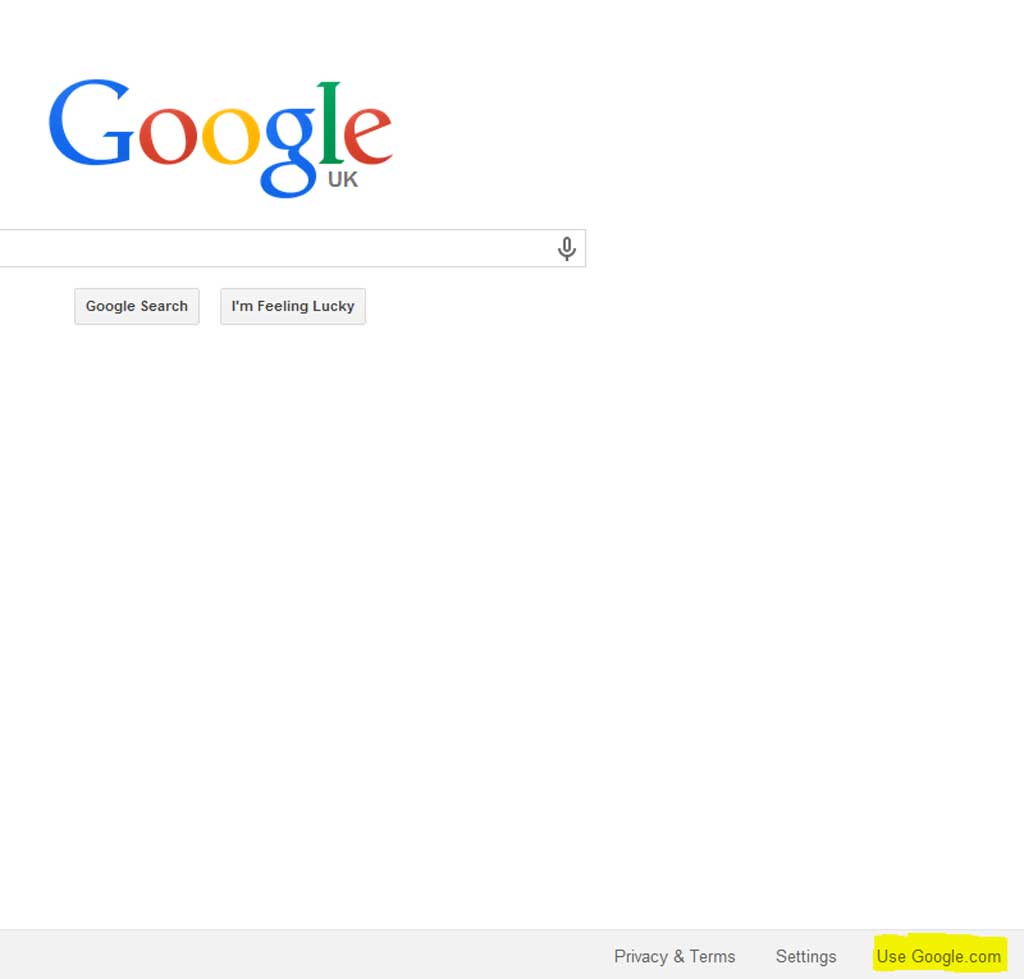The image depicts a section of the Google homepage on a white background. Dominating the left side is the iconic Google logo, composed of a large blue capital 'G', followed by lowercase letters: a red 'o', a yellow 'o', a blue 'g', a green 'l', and a red 'e'. Just below the letters 'l' and 'e', in light grey, is the country designation "UK".

Centrally positioned on the page is the familiar search bar, white with a light grey border, designed for users to enter their queries. Adjacent to the right end of the search bar is a microphone symbol resembling a pill, with a small letter 'C' beneath it, indicative of voice search capability.

Beneath the search bar are two clickable buttons in mid-grey with a darker grey border, featuring dark grey or black text. The first button reads "Google Search" and the second button reads "I'm Feeling Lucky".

At the bottom of the image, there's a banner in mid-grey containing options with dark black or dark grey text. It reads "Privacy and Terms" followed by "Settings". Additionally, there is a highlighted section below that saying "Use google.com," emphasized with a yellow background.

The image appears slightly truncated on the left side, partially cutting off the search bar.